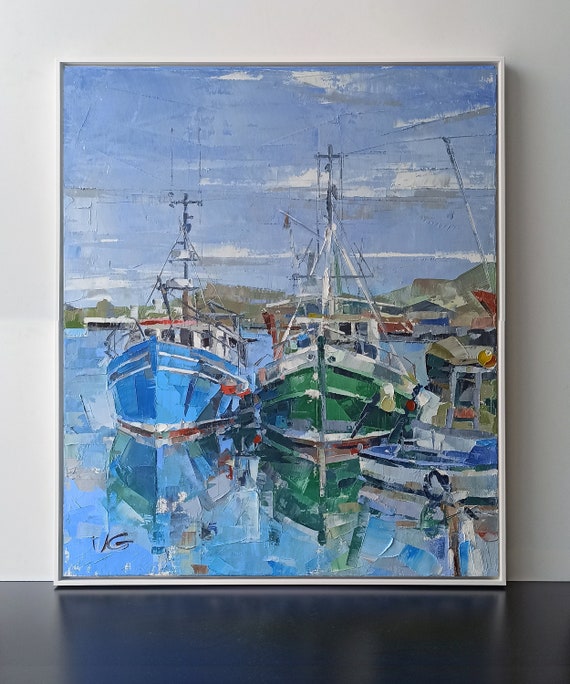This detailed painting, which is taller than it is wide and framed in white, captures a vibrant seaside shipyard scene. Prominently displayed against a white wall and touching a black floor, the artwork features two main vessels: a blue yacht-style boat with tall masts and four windows on the left, and a green boat of similar style but with a slightly taller mast on the right. Next to the green boat, partially visible on the far right, is a smaller tugboat with a blue top and white bottom. The blue and green hues dominate the pallet, with the artist's expressive paint strokes capturing the boats' reflections in the crystal blue water beneath them. In the background, serene green mountains rise under a light blue sky dotted with white clouds, completing the harmonious maritime scene. The artist, whose initials "VG" are signed in the lower left corner, has rendered this scene in an abstract oil painting style, emphasizing the tranquil yet vibrant essence of a bright, sunny day on the water.